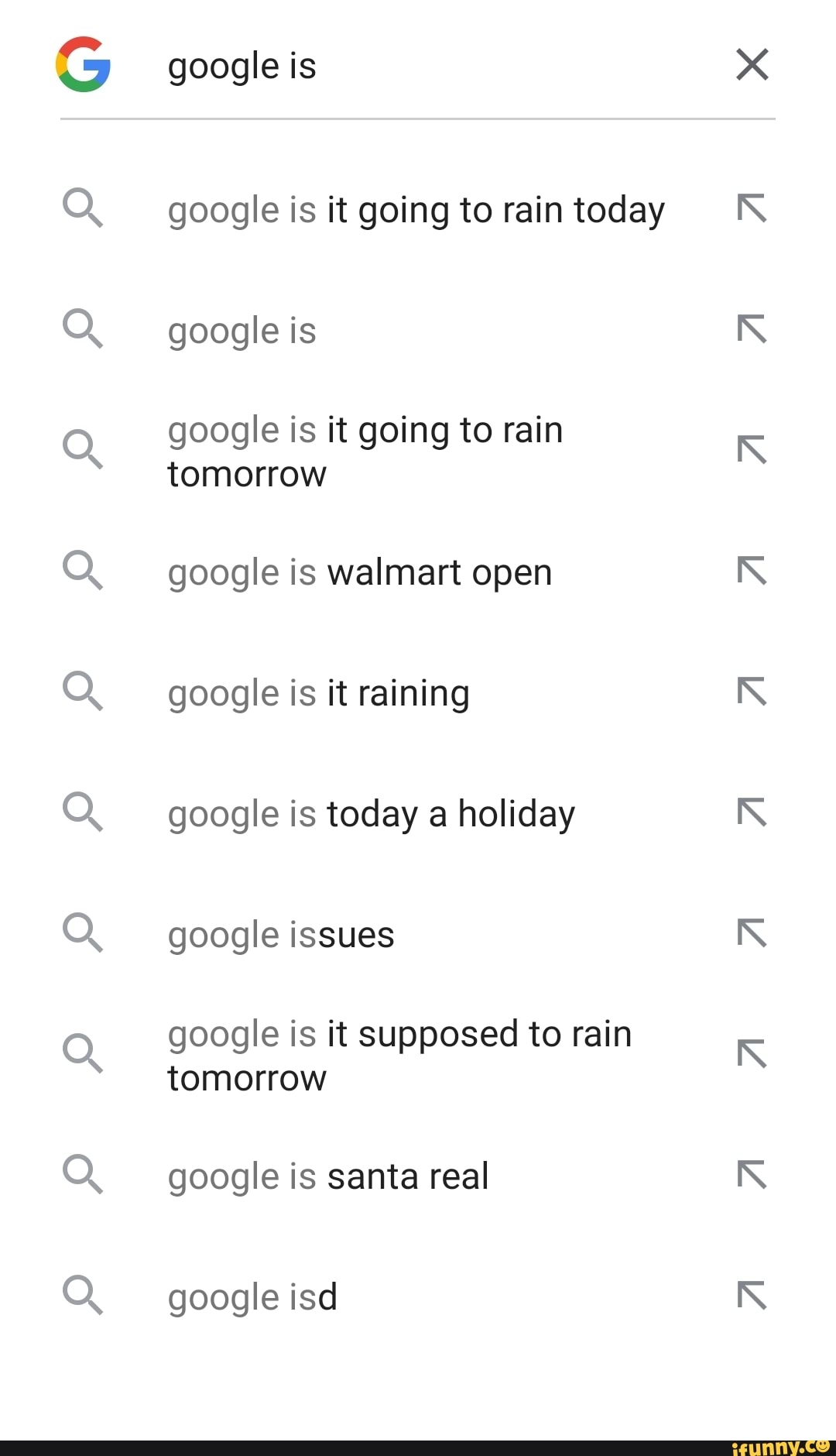In the top left corner of the image, there is a white background with the Google logo prominently displayed. The logo consists of a multicolored capital "G" that transitions from red to yellow, then green, and finally blue. To the right of the logo, the words "Google is" are typed in black text, accompanied by a gray "X" icon and an underlined search bar. 

Each suggested search result below the bar begins with a gray magnifying glass icon on the left and a gray arrow pointing diagonally to the left on the right side of the text. The suggestions are auto-completions that Google often generates. Each one starts with "Google is" in gray, followed by the rest of the query in black. The auto-completed search queries are as follows:

1. "Google is it going to rain today?"
2. "Google is it going to rain tomorrow?"
3. "Google is Walmart open?"
4. "Google is it raining?"
5. "Google is today a holiday?"
6. "Google issues" (with "is" in gray and "sues" in black)
7. "Google is it supposed to rain tomorrow?"
8. "Google is Santa real?"
9. "Google ISD" (with "IS" in gray and "D" in black)

The gray colors of the magnifying glass icons, arrows, and parts of the text provide a consistent visual theme across the suggestions on the search interface.